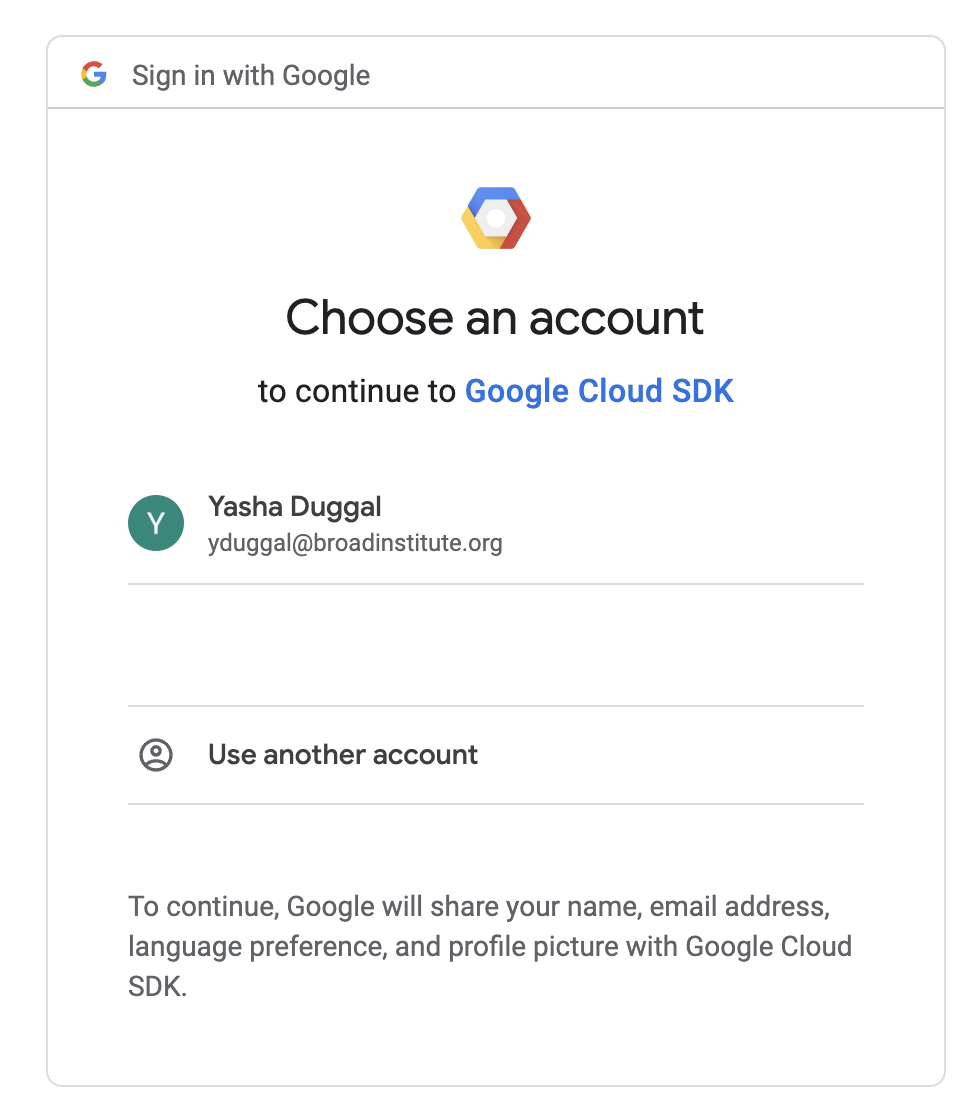The image displays a Google sign-in interface for accessing the Google Cloud SDK. At the top, there is a notification prompting the user to "Sign in with Google." Below it, the message "Choose an account" is displayed. The Google logo appears in an unconventional design, depicted as a hexagon with yellow and red segments. Users are asked to select an account to proceed, with the first option shown as a green circle containing a white "Y," representing the account of Yasha Dugal, whose email is ydugal@broadinstitute.org. There is also an option to sign in with a different Google account. The notification informs the user that by continuing, Google will share their name, email address, language preference, and profile picture with the Google Cloud SDK. This sets up the expectation that further verification steps may be required after selecting an account.